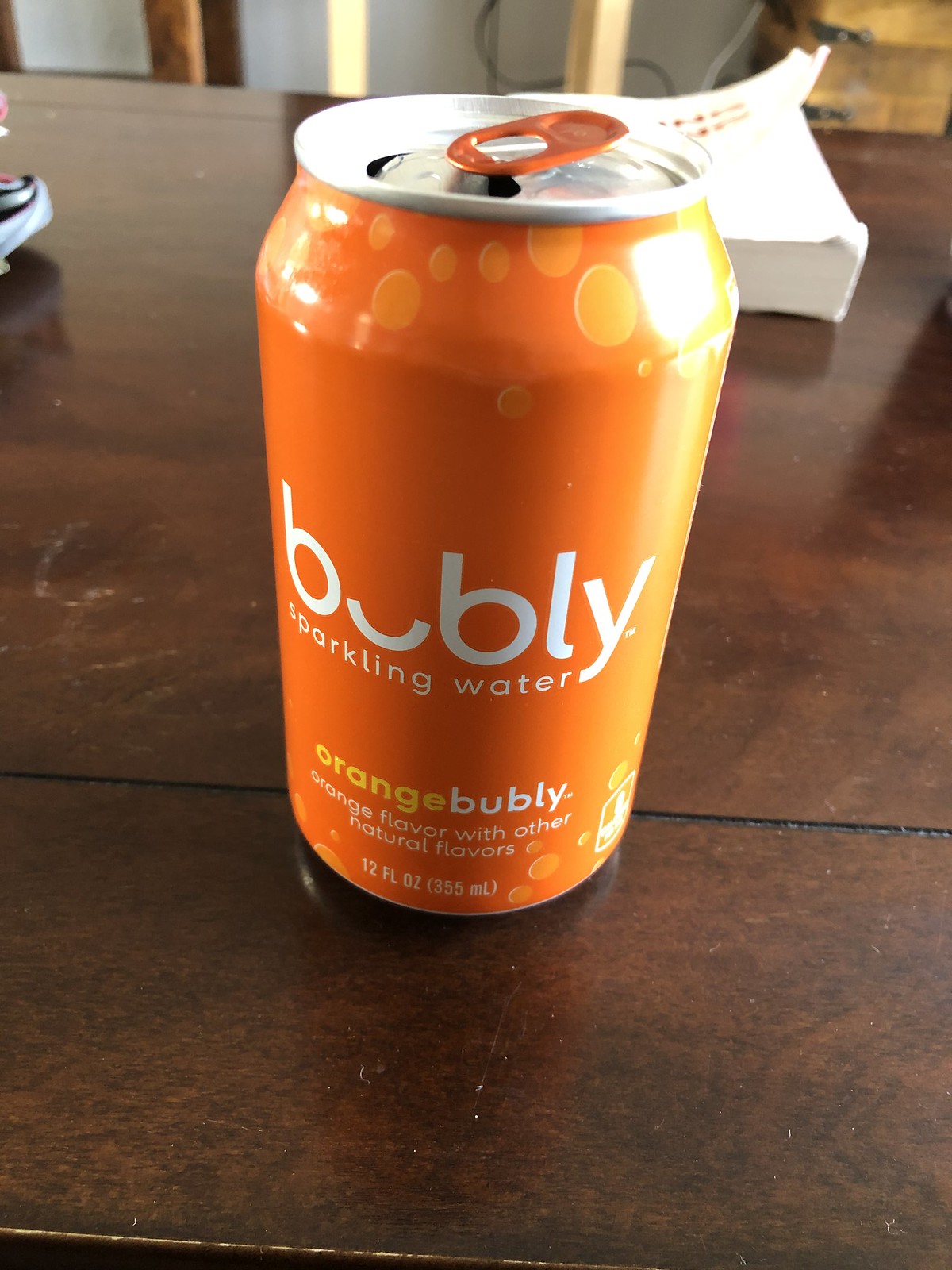The image features a can of sparkling water prominently displayed on a dark brown, aged wooden table, which dominates the lower portion of the picture. The table bears lighter marks and scratches, indicating its wear and age. In the background, a thick white book is visible, though its title or content remains obscured due to the bright reflection off its pages.

The can itself is vibrant with an orange color palette, complemented by lighter orange bubbles that suggest the effervescence of the drink within. The top of the aluminum can is silver, with a distinctive bright orange pull-tab, indicating the can has been opened, as evidenced by the black area visible in the opening. 

The can is decorated with white text, prominently reading "bubly" (stylized as B-U-B-L-Y) and labeling the drink as "sparkling water." Below it, the text specifies "orange bubly" in orange font, further clarifying that this is an orange-flavored beverage. Additional text in white mentions "orange flavors with other natural flavors" and specifies the volume as "12 fluid ounces."